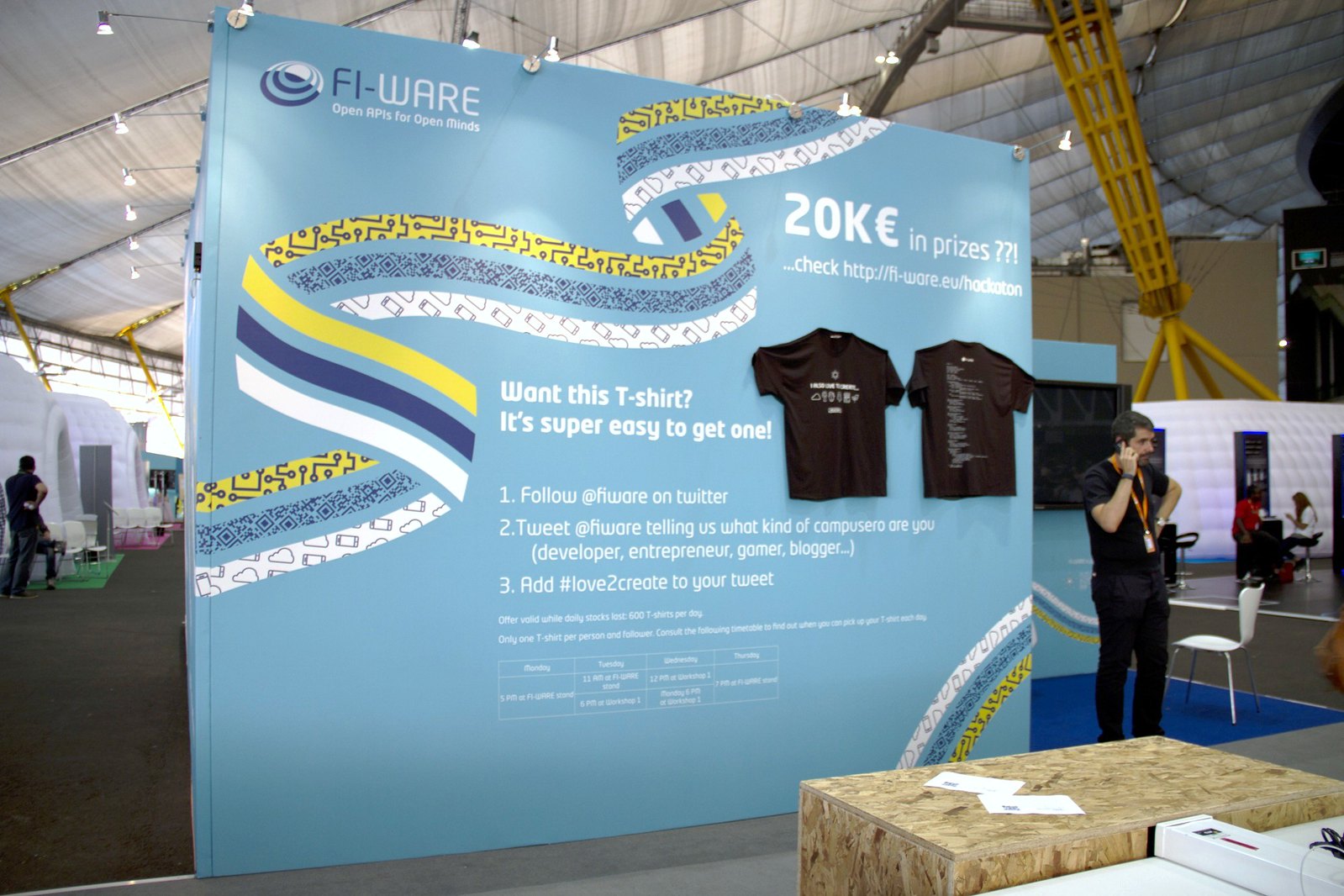The photograph captures a vibrant scene inside a convention hall. Dominating the right side of the image is a man dressed entirely in black, adorned with an orange lanyard, and engaged in a phone conversation. He stands beside a large light blue sign featuring a prominent three-stripe ribbon in white, blue, and yellow, winding from the lower left to the top right. The sign advertises "20K in prizes" and provides details about a website, inviting attendees to participate in a t-shirt giveaway by following FIWARE on Twitter, tweeting their profession (e.g., developer, entrepreneur, gamer, blogger), and using the hashtag #LoveToCreate. Two black t-shirts are stapled to the sign, displaying white text with instructions for the giveaway. The convention hall itself is bustling with activity; people are seen conversing, seated on white chairs or standing. The area features a mix of gray, pink, and green carpets, with structural elements like white ceilings, a yellow slanted beam, and various other fixtures contributing to the dynamic atmosphere.